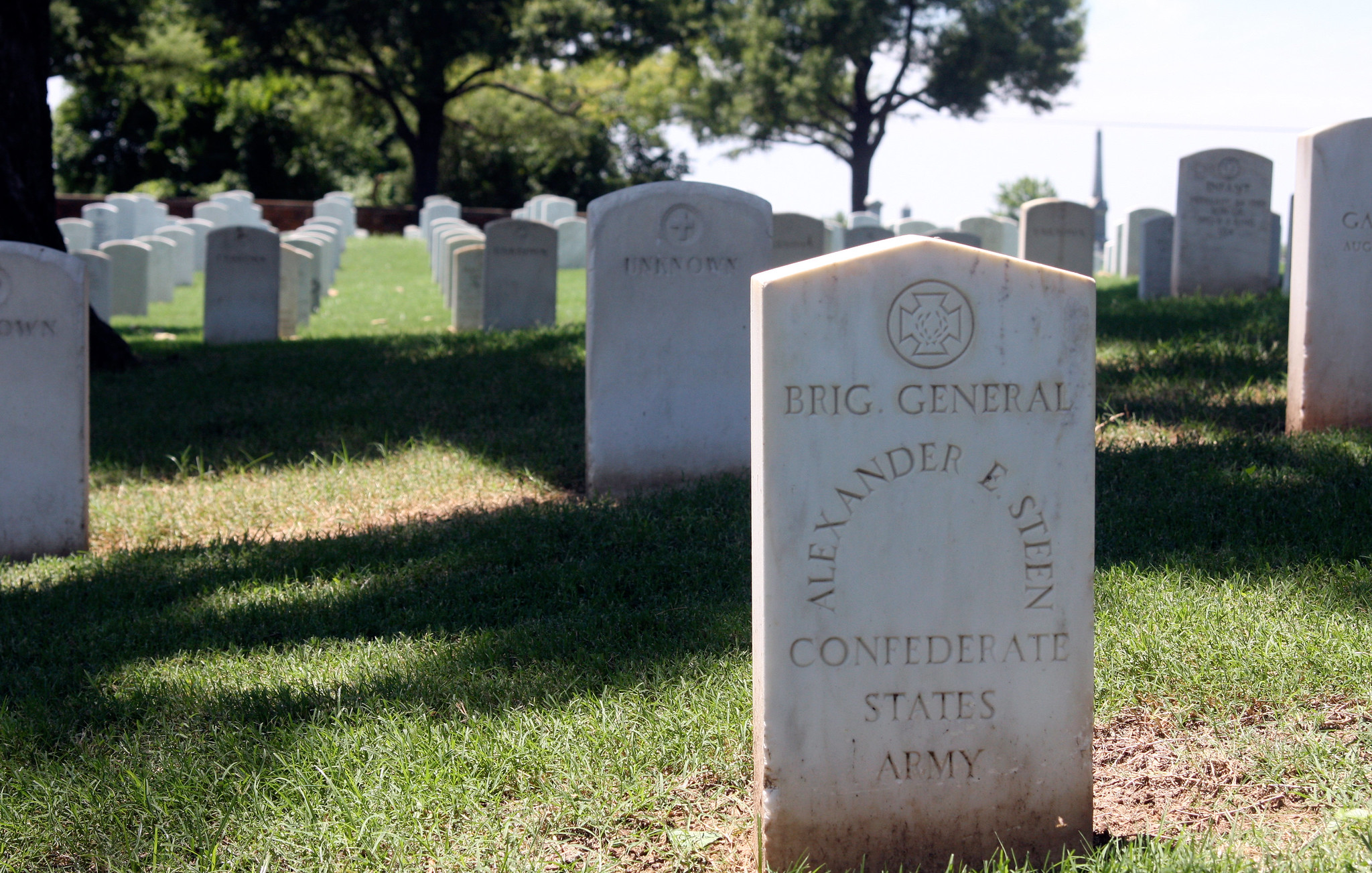The image captures a serene cemetery with uniform headstones arranged meticulously in rows on a neatly mowed field. The sun casts shadows through the green foliage of large oak trees, adding a touch of tranquility. Dominating the foreground is a prominent tombstone inscribed with "Brigadier General Alexander E. Steen, Confederate States Army," devoid of dates, and surrounded by freshly disturbed dirt, suggesting recent placement. Behind it stands a subtler marker bearing a cross, faintly readable, indicating an "UNKNOWN" interred soldier. A possible church steeple emerges in the distant background, affirming the solemn atmosphere of this well-planned Confederate Army burial ground.